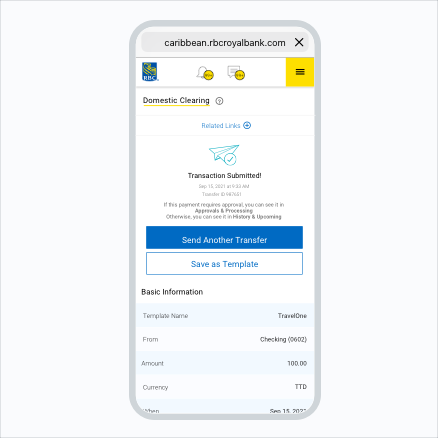This detailed descriptive caption outlines the contents of an image, providing a comprehensive visual description of a smartphone screenshot. Here is the cleaned-up and enhanced caption:

---

This image captures a screenshot from a smartphone, clearly outlining the device's display. The background of the page is white, while the outer frame of the smartphone is gray. At the top of the screen, within a gray rectangle, the web address “caribbean.rbcroyalbank.com” is prominently displayed.

The top border features the Royal Caribbean Bank logo on the left, and on the right, a yellow square containing three horizontal black lines indicates a drop-down menu. Centrally located, there is a notification bell icon accompanied by a yellow circle, as well as a live chat icon with a similar yellow circle.

Beneath this top border, the text "Domestic Clearing" is clearly visible, next to a light blue paper airplane icon. Below, the message "Transaction Submitted" is displayed, although the following smaller text is illegible. Two button options are clearly distinguishable: a blue rectangle with "Send Another Transfer" in white text, and a white rectangle with "Send As Template" in blue text.

Further down, there is a section labeled "Basic Information" in black font. Under this section are the following details:
- Template Name: travel1
- From: Checking
- Amount: $100
- Currency: TDD

There is an attempt to show the date, but only partially visible text suggests it might be “September 15th, 2023,” though the year is cut off and not entirely clear.